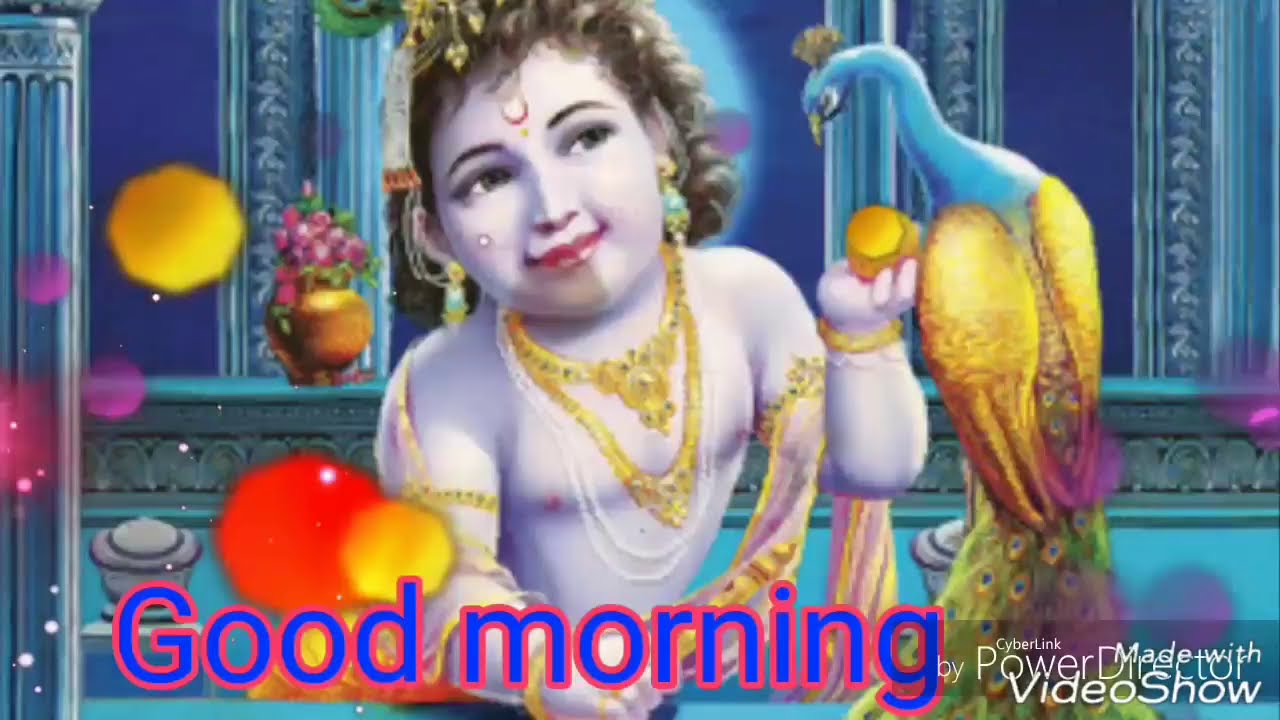The image is a vibrant, artistic depiction of a Hindu deity, portrayed as an effeminate-looking man with blue skin, dressed in many gold necklaces, and adorned with red lipstick. He has curly hair, a crescent marking on his forehead, and a warm, smiling expression. Sitting beside him is an exotic bird, resembling a peacock, with a blue neck and head, golden wings, and green tail feathers. The scene is set against a blue-domed wall with intricate arches, and additional elements include a stone ledge adorned with a gold vase and pink flowers, as well as floating purple and yellow orbs, giving the overall composition a mystical and ethereal feel. At the bottom of the image, text in blue and red letters states "good morning," while the lower right-hand corner is marked with "by CyberLink PowerDirector," overlaid with "made with video show."